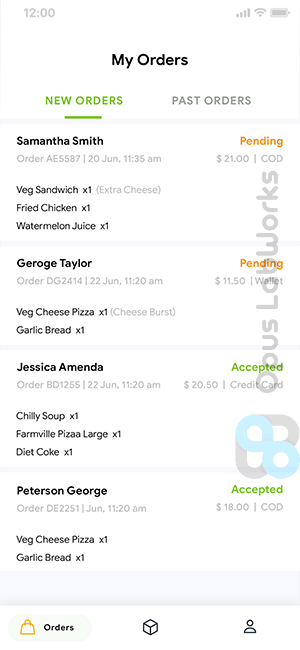**Image Description:**

In the center of the image, we see various food and drink items, as well as details of multiple food orders highlighted with their respective statuses.

- **Samantha Smith:** Placed an order costing $21, which includes a vegetable sandwich, fried chicken, and watermelon juice. 
- **George Taylor:** Made an order costing $11.30. The details mention a vegetable pizza and garlic bread, but the status indicates the garlic bread is still pending.
- **Jessica Amanda:** Accepted an order that includes chili soup, a large Farmville pizza, and one diet coke, totaling $20.50.
- **Peterson George:** Accepted an $18 order consisting of a vegetable pizza and one garlic bread.

On the screen, we can also see various tabs and options like "cube profile," "new orders," "past orders," and "my orders," which are organized neatly. The timestamp is noted at "12 in," demonstrating it’s set in time zone information located at the top left. Additionally, there’s data about "Wi-Fi," "battery," and "gray" notifications on the top right.

At the bottom of the screen, there’s a quirky personal message or audio tag possibly playing: "They call me Dr. Worm. Good morning, how are you? I'm Dr. Worm. I'm interested in things. I'm not a real doctor, but I am a real worm. I am a natural worm. I live like a worm. I like to play the drums." This adds an interesting, whimsical touch to the image.

Overall, the image reflects a snapshot of food orders with a mix of itemized details and a playful, unexpected element.